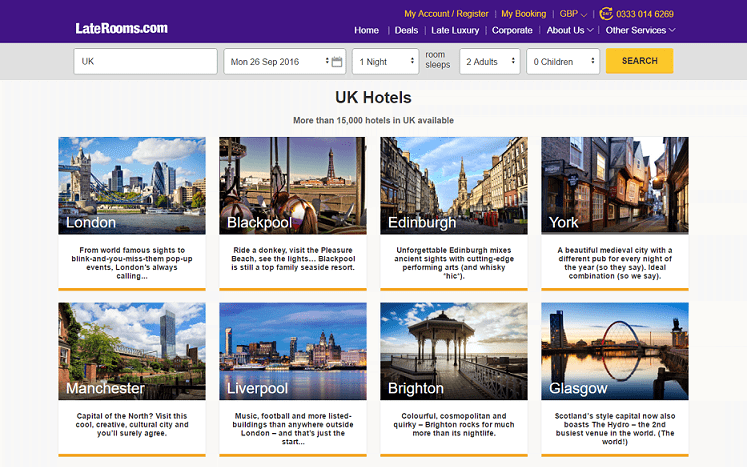The image displays the Laterooms.com website. At the top of the page, there is a blue banner with the website name "laterooms.com" prominently displayed in white text. Below the banner, a navigation bar features various links in white, including "Home," "Deals," "Late Luxury," "Corporate," "About Us," and "Other Services."

In the center of the page, a headline reads, "UK hotels, more than 15,000 hotels in the UK available." Below this headline, there are eight images portraying different cities, each with the city's name in the lower left corner of the image. The cities featured are London, Blackpool, Edinburgh, York, Manchester, Liverpool, Brighton, and Glasgow.

The leftmost image shows London. Beneath it, the caption reads, "From world-famous sites to blink-and-you-miss-them pop-up events, London is always calling." Next to London, the image of Blackpool includes a caption that says, "Ride a donkey, visit the Pleasure Beach, see the lights. Blackpool is still a top family seaside resort." The image featuring Edinburgh has a caption that reads, "Unforgettable Edinburgh mixes ancient sites with cutting-edge performing arts and whisky."

Each city image provides a glimpse of what visitors can expect, highlighting key attractions and unique experiences that make these destinations special.